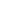In this indoor New Year's Eve party scene, a lively group of friends is posing for a festive photo. The setting appears to be a bar, dimly lit with a flat-screen TV partially visible in the background. The group is a mix of men and women, all smiling and clearly enjoying the celebration. 

On the left side, a man with black hair, wearing a black jacket, is flashing the peace sign. Next to him is a girl with black hair and a matching black jacket. Two other girls, both in black dresses and also with black hair, are wearing colorful "Happy New Year's Eve" headbands, one pink and one green.

On the far right, there's a man sporting a black blazer over a black sweater, and another man in a tie and white collared shirt who is also wearing glasses and smiling brightly. 

They are all gathered around a black table strewn with clear plastic cups filled to the top with drinks, some adorned with lemon wedges and black straws. The atmosphere pulses with the excitement of the New Year, as indicated by the festive attire and happy expressions of everyone in the photo.